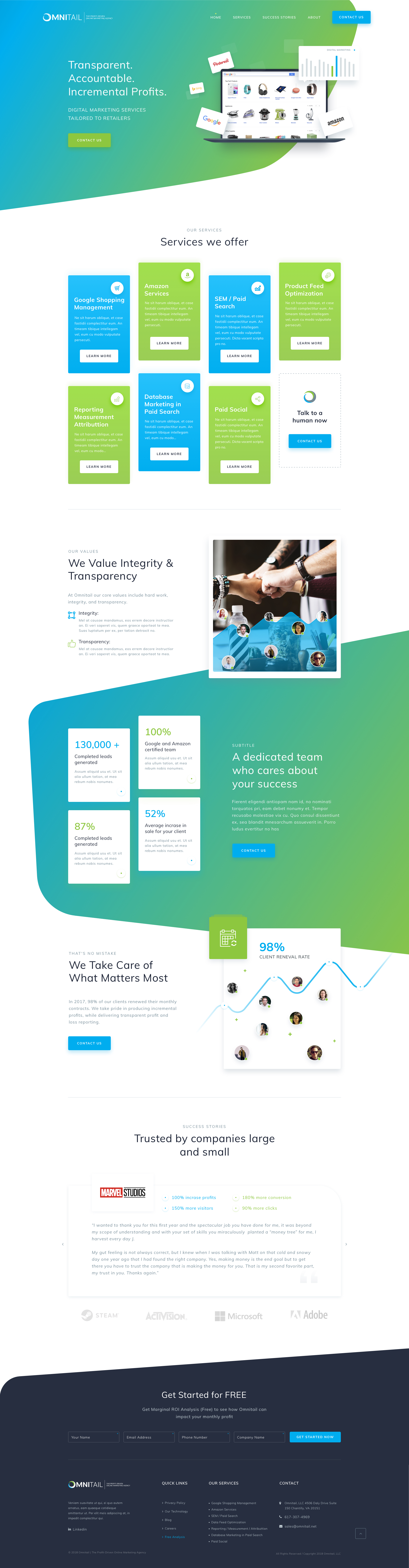The image appears to be a highly compressed screenshot of a website, making it difficult to discern fine details. 

**Top Section:**
- **Background:** The top section features compressed graphics.
- **Headers:** Small, white letters are spread across the top. 
- **Main Text:** The central text reads, "Transparent, Accountable, Incremental Profits," accompanied by smaller white text.
- **CTA Button:** A green clickable tab is present.

**Central Section:**
- **Image:** To the right, there is an image of a computer monitor with a black border and white interior, including small tabs around its sides.
- **Text:** "Services We Offer" is prominently displayed in the middle of a white background.
- **Squares with Info:** 
  - A blue square with information.
  - Followed by alternating blue and green squares, each with white letters and a clickable tab labeled "Learn More" in black text. 
  - Another sequence of green and blue squares is underneath, culminating with a white square that says, "Talk to a Human Now" and a blue tab labeled "Contact Us."

**Left Side:**
- **Text:** Under a statement, "We value integrity and transparency," additional information is provided.
- **Image:** Adjacent to this text is an image of three people bumping fists.

**Bottom Section:**
- **Color Scheme:** A gradient border starts with blue on the left and transitions to green on the right.
- **Stats:** Four white squares on the left, arranged in a 2x2 grid, feature large numbers in the top left corners and percentage values with text underneath.
- **Text Block:** To the right, a message reads, "A dedicated team who cares about your success," followed by a paragraph and another blue "Contact Us" button.
- **Tabs and Bar:** Tabs for further navigation are spread across a white background. 
- **Footer:** A prominent black bar at the bottom holds more text and additional clickable tabs.

Overall, the webpage emphasizes transparency, accountability, and customer engagement through a mix of informative sections, visual elements, and call-to-action buttons.